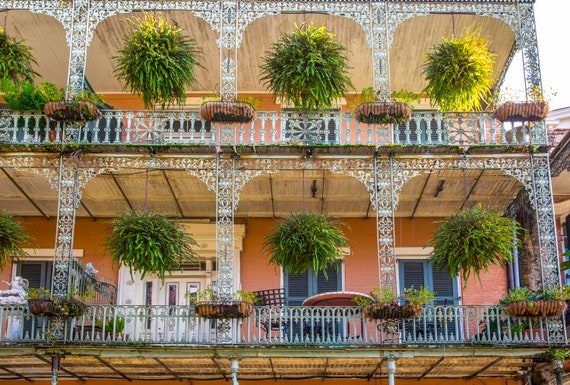This image showcases a charming, retro-style building that resembles a small hotel or vacation rental. The structure features two levels, each with its own spacious balcony adorned with decorative filigree lattice columns and elegant wrought iron arches. The building’s exterior is painted in a distinctive pastel pink hue, complemented by old-style orange accents, and is framed with silver scaffolding. Evergreen fern-like plants hang gracefully from the balconies, nestled between each window and column, adding a lush green contrast to the facade.

White, double doors provide access to the balconies, flanked by vibrant, dark blue window shutters with white framing. On the lower balcony, there are tables and chairs positioned next to the doors, inviting relaxation and leisure. The overall architectural style evokes a blend of Art Deco and French Quarter charm, reminiscent of buildings found in the southern United States, notably around New Orleans. This picturesque setting combines vintage aesthetic with tropical greenery, creating a warm and inviting atmosphere.